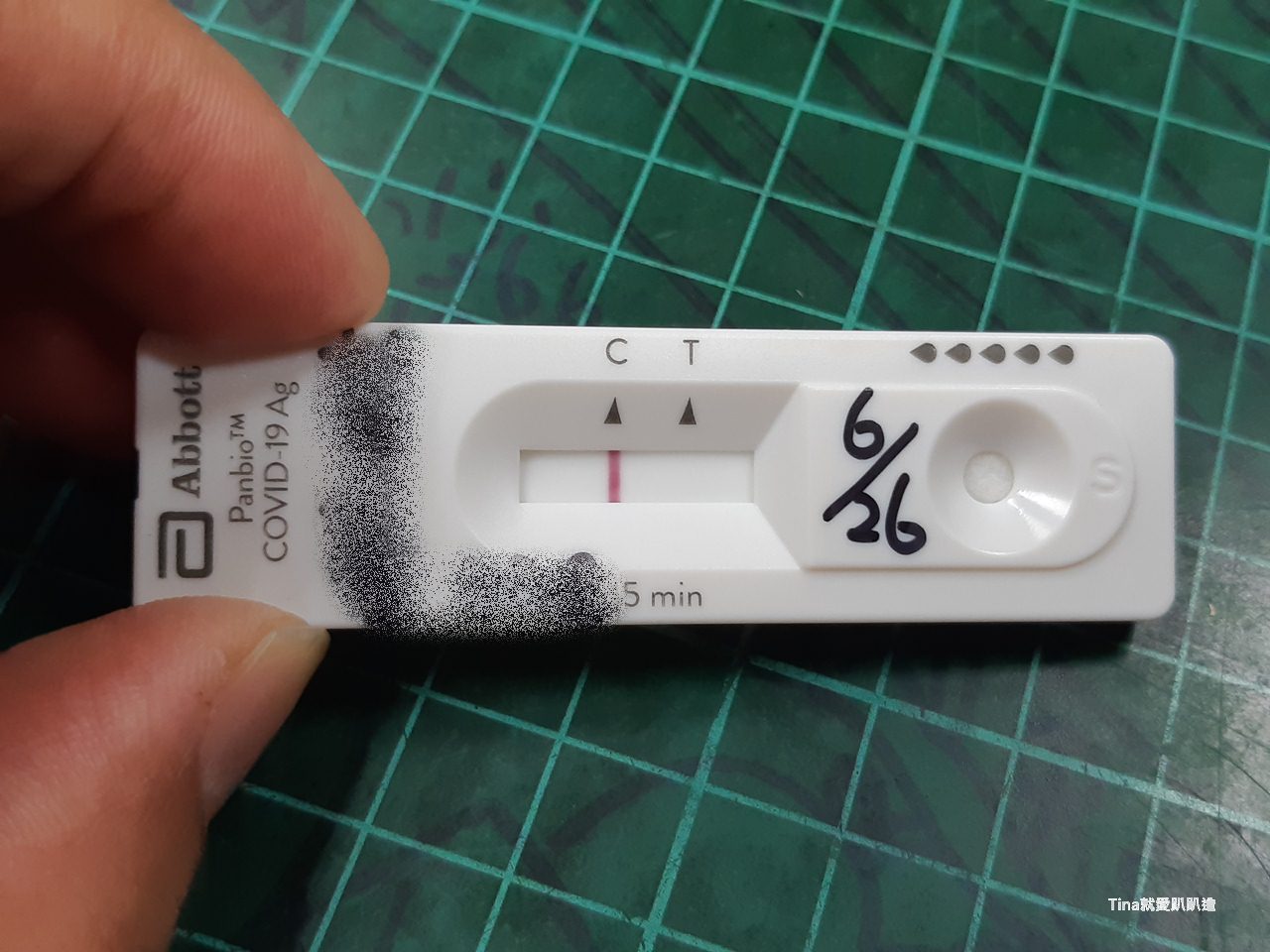The image is a close-up, color photograph of a small, rectangular COVID-19 antigen test placed on a green, tiled countertop with green grout lines. The test device, branded with the "Abbott" logo, prominently displays "COVID-19 AG" on its left side. There is a black smear, likely decorative, across the surface of the test. 

At the center of the test kit is a narrow window showing the test results, with markings "C" and "T". The "C" position has a red line, indicating the result. On the right side of the test, a small depression acts as an application area, featuring an illustration of five blood droplets, not real but highlighted as part of the design to indicate the area for sample collection. A date, "6/26", is handwritten on the device in black marker, possibly indicating the date the test was taken.